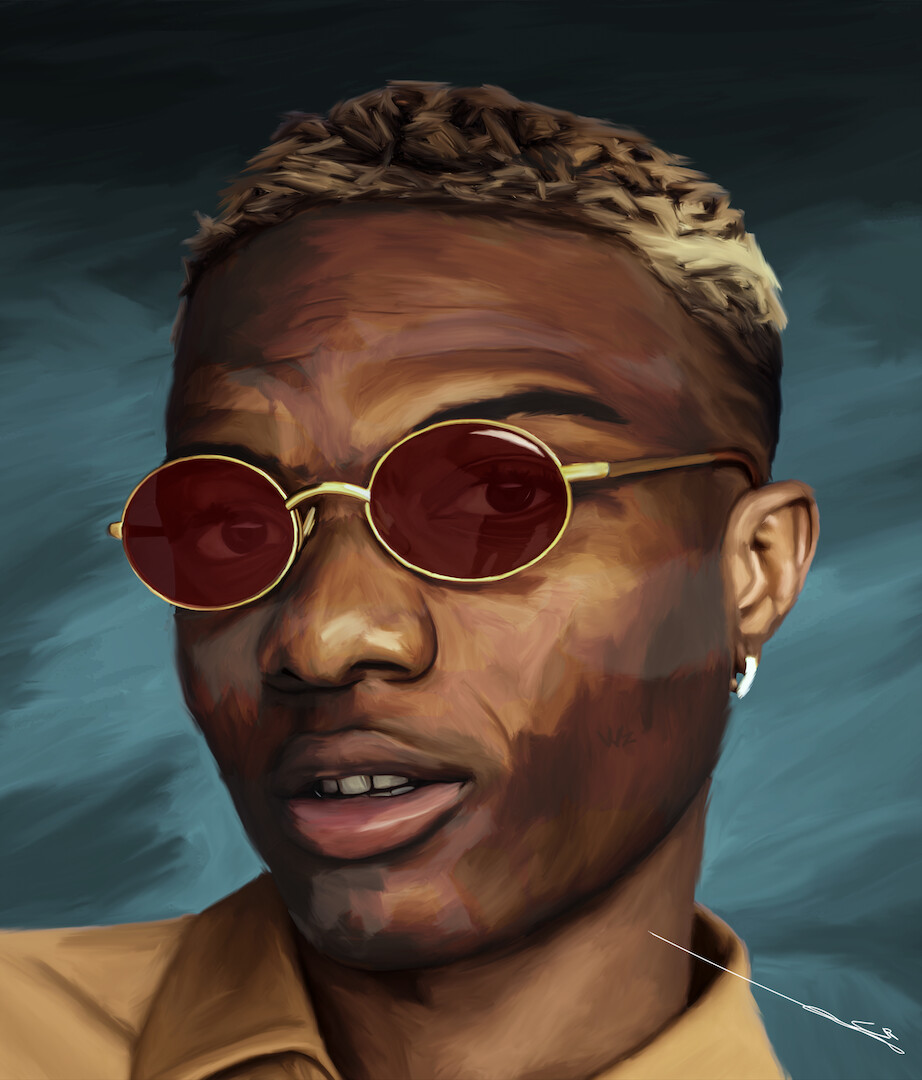This detailed artist's rendering portrays a young African-American male with a distinctive appearance. His complexion is a mix of brown and tan hues, and he sports dark hair accentuated with either blonde highlights or black strands, adding an intriguing texture to his look. His eyebrows are black, and his lips are a pinkish color, partially open to reveal his white teeth. The man is wearing stylish gold-toned round sunglasses with red lenses, highlighted by black and brown frames. His left ear features a noticeable hoop earring. He is dressed in a light tan, button-down collared shirt. The background is a slate blue with darker gray and white shades, creating a dynamic and artistic backdrop. This portrait appears to have a filter applied, giving it a painted, liquefied effect. A signature, though not legible, is placed in the lower right-hand corner at a triangular angle.